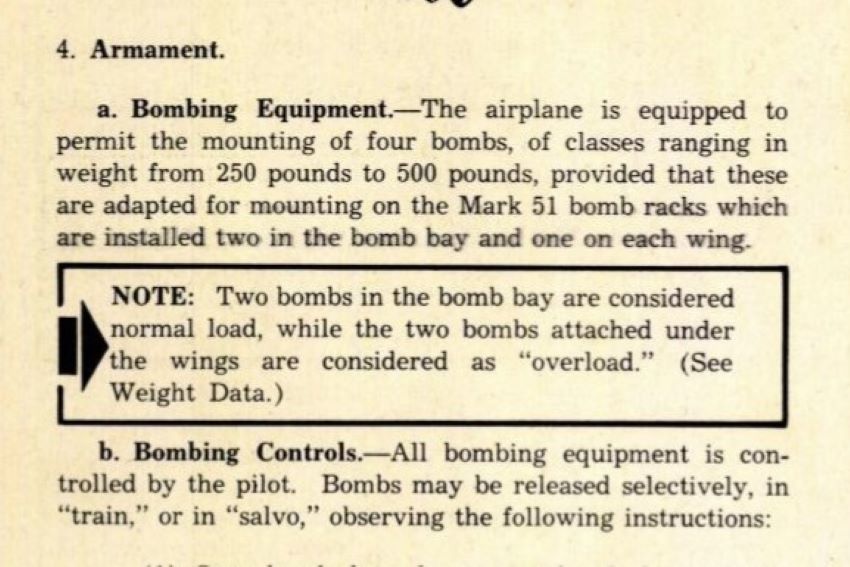This excerpt appears to be a detailed and slightly aged black and white print, possibly from a military manual or brochure, with a discolored white background bearing a slight pink hue. It outlines the fourth point under armaments, with a specific focus on bombing equipment and controls. The section labeled "A. Bombing Equipment" describes the airplane's capability to mount four bombs, each ranging from 250 to 500 pounds, on Mark 51 bomb racks—two located in the bomb bay and one on each wing. A rectangular box notes that while two bombs in the bomb bay constitute a normal load, the two bombs mounted under the wings are considered an overload, referencing weight data for further detail. Subsequently, under the heading "B. Bombing Controls," it specifies that all bombing equipment operations fall under the pilot's control, allowing bombs to be released either selectively "in train" or in "salvo," with instructions to follow.